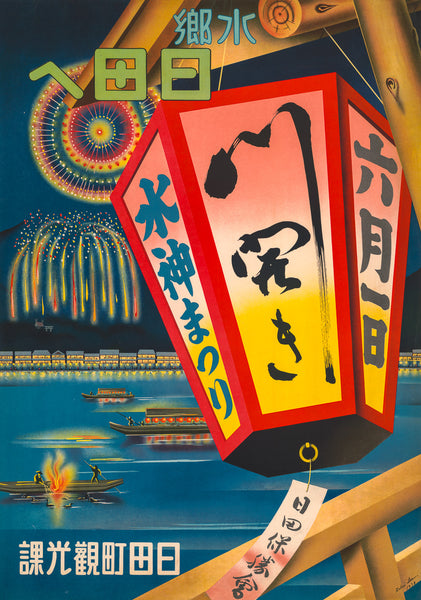This vibrant poster, likely for a Chinese event, prominently features an intricately designed Chinese lantern as its centerpiece. The hexagonal-prism lantern, with a larger top than bottom, boasts a red wooden frame and translucent sides shaded from red to yellow. Chinese characters adorn the lantern's three visible sides, which are blue on the left, black in the middle, and gray on the right. Hanging from a bamboo post in the foreground, the lantern is part of a detailed illustration rather than a photograph, rendered in a vivid pop art style.

Surrounding the lantern is a wooden railing, also in a bamboo color, which enhances the scene's richness. In the foreground, a flat, blue river reflects three boats, each with stick-figure occupants. The closest boat harbors a fire, while the other two are illuminated by lights. Behind the water, a distant shoreline is dotted with tiny, lit-up buildings.

The night sky, a gradient of dark blue, indigo, and black, is alive with stylized, rainbow-colored fireworks. A large circular firework with red, blue, and yellow dots spreads its vibrant lines across the sky. Below, sparkles of white, yellow, and red light cascade like a waterfall, adding a dynamic flair to the background, which may also hint at a mountainous landscape obscured by the pyrotechnic display. This compelling, festively illustrated poster, possibly for a New Year celebration, is a captivating blend of traditional motifs and modern artistic expression, completely adorned with Chinese characters.